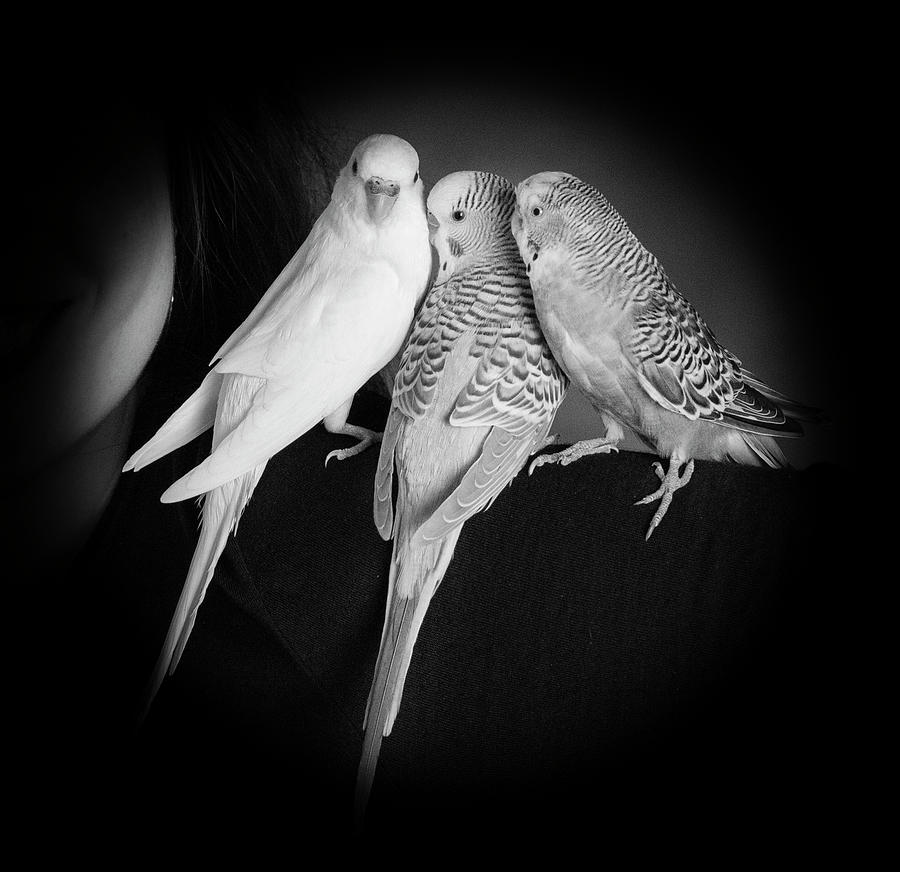In this detailed black-and-white photograph, set in a square format, three parakeets are perched closely together on the left shoulder of a smiling woman. The image, predominantly dark with the main light focus on the birds, partially obscures the woman's face, leaving glimpses of her dark brunette hair visible as it hangs at least shoulder length. The woman, whose face is relegated to the side and partially shrouded in shadows, is attired in what appears to be a suit jacket or a black shirt. Of the three birds, the leftmost parakeet is uniformly light-colored with small black eyes. The middle parakeet, displaying a distinctive striped pattern across its wings and body, nestles affectionately into the bird on its left. Similarly patterned, the rightmost parakeet's detailed claws firmly grasp the fabric of the woman's clothing as it gazes off into the distance. The backdrop is a black fabric, further accentuating the illuminated trio of parakeets in delicate repose on the woman's shoulder.